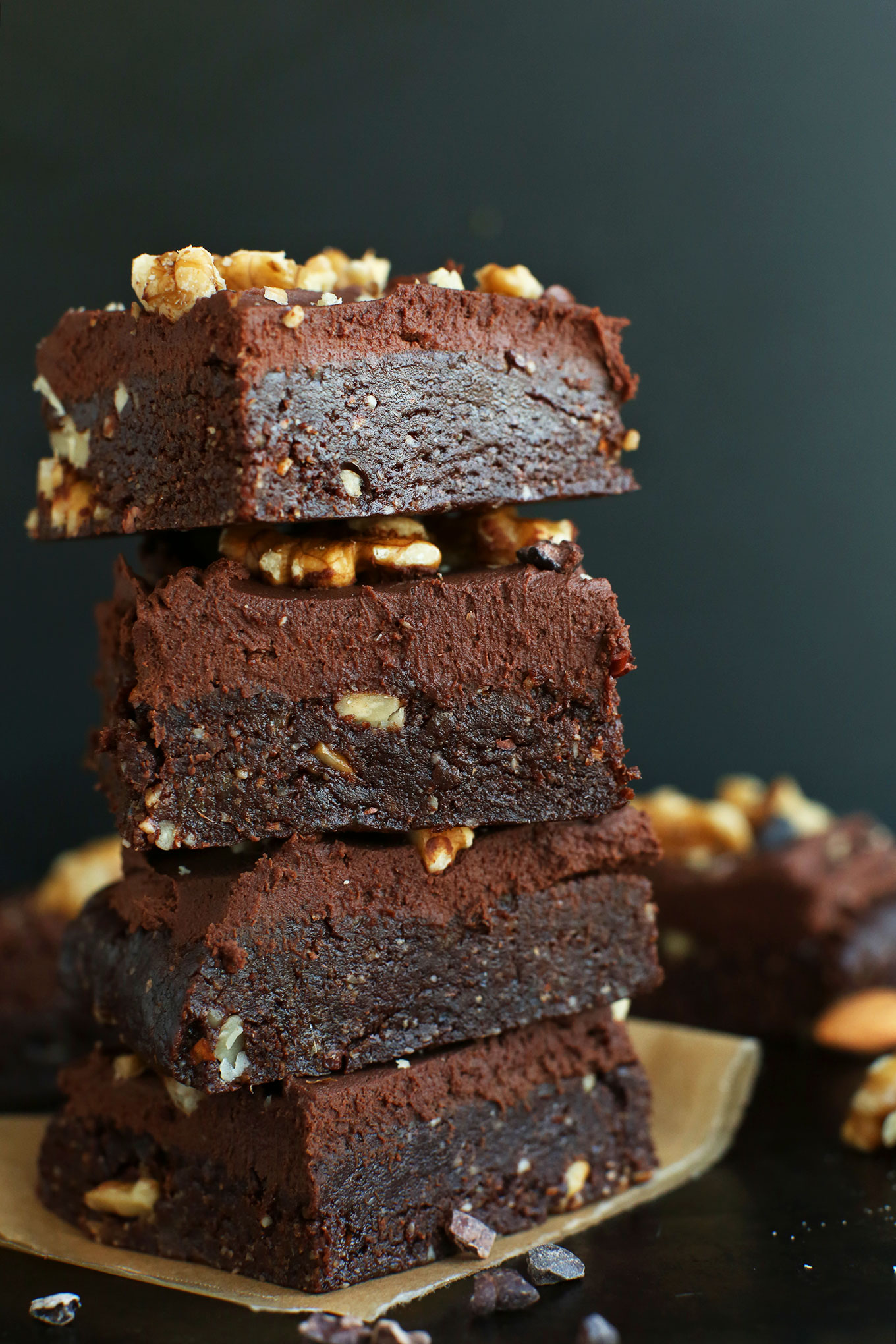In this detailed photograph, four rich and indulgent brownies are stacked neatly atop each other, presenting a deliciously tempting sight. Each brownie is cut into a rectangular shape, broader and longer than it is thick, with a darker, fudgier layer forming the base of each piece. Atop this dense layer lies a thinner, lighter brown, more porous layer, suggesting either a lighter chocolate or possibly an icing. The surface of each brownie is adorned generously with walnut pieces, and occasionally, smaller bits of walnut appear to be baked into the brownies themselves. The stack of brownies rests on a slightly elevated, square paper plate, turned up on two sides, enhancing its presentation. This paper plate sits on a black-colored tabletop or countertop, with more indistinct brownies visible in the blurred background, suggesting a setting filled with these delectable treats. Tiny white flakes, perhaps coconut, are scattered in front of the brownies, adding an extra layer of texture and visual interest to the scene. The light gray wall in the background provides a neutral backdrop that makes the rich tones of the brownies stand out even more.